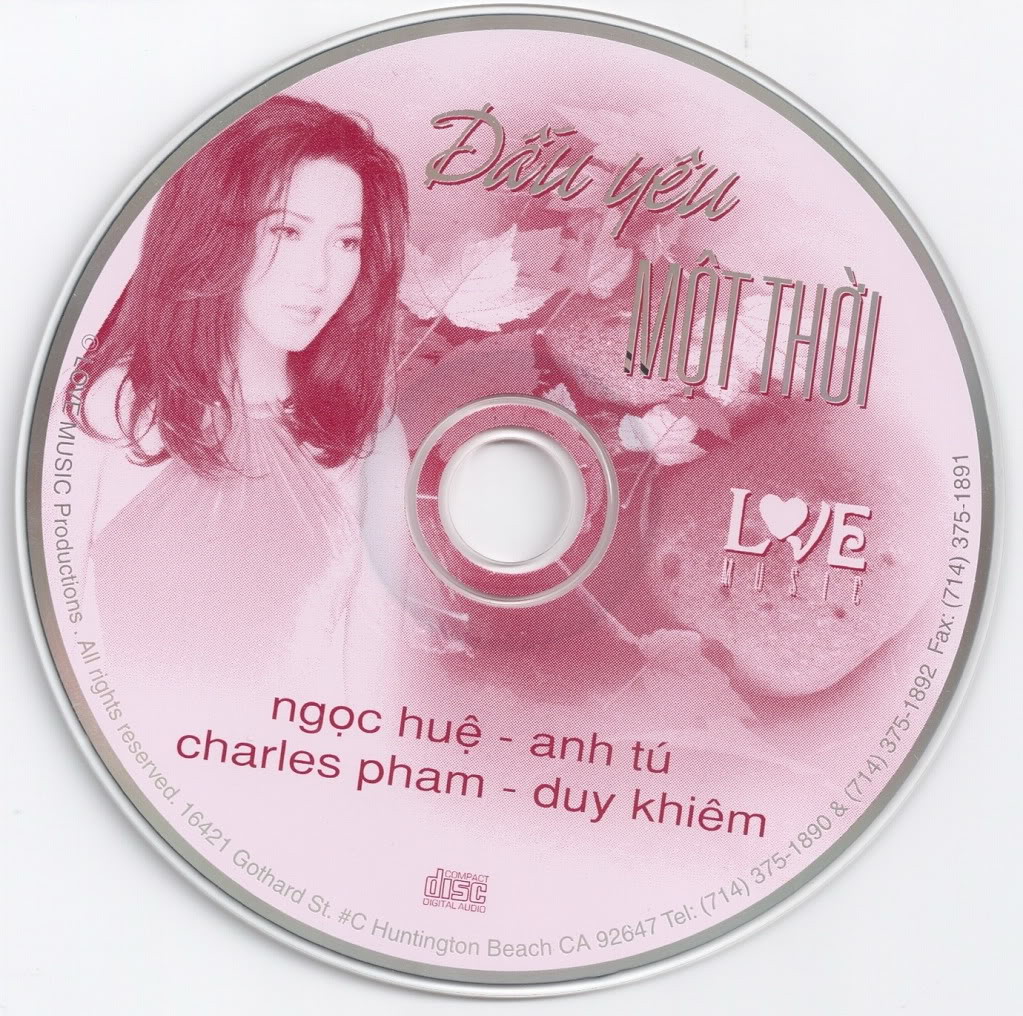This image features a CD with a prominent photograph of a young Asian woman named Dayu Montthoi, who has long hair and is dressed in a sleeveless, neck-halter dress in shades of pink and gray. The CD is pink with a background that includes floral elements and rocks. The title "Love Music" is displayed below a title in Vietnamese, which supports that the text on the CD is primarily in the Vietnamese language. The left side of the CD features the woman's photograph, while the right side displays several names: Ngoc Hue, Anh Tu, Charles Pham, and Dai Kim. Surrounding the edge of the CD are the words "Something M Music Productions, All Rights Reserved," along with their address at 16421 Gothard Street, number C, Huntington Beach, California, 92647. Additionally, contact details include phone numbers 714-375-1890 and 714-375-1892, and a fax number 714-375-1891.